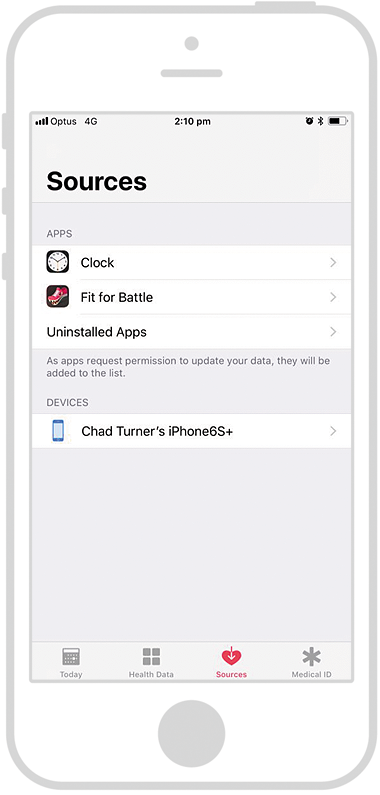Screenshot of an iPhone displaying the "Sources" section of the Health App. The image includes the iPhone's bezel in a white design. 

At the top left corner:
- Four bars of signal strength.
- Connected to the Optus network.
- 4G connectivity.

In the middle of the status bar:
- Time displayed as 2:10 PM.

In the top right corner:
- Alarm clock symbol indicating an active alarm.
- Bluetooth symbol indicating Bluetooth is on.
- Battery level at approximately 50%.

Main Content:
- Heading: "Sources."
- Below the heading, there is an "Apps" section with two listed applications:
  1. Clock - a time management application.
  2. Fit for Battle - likely a video game.
- Below the listed apps, there is an "Uninstalled Apps" option.

Navigation:
- Each option (Clock, Fit for Battle, and Uninstalled Apps) includes a right arrow leading to a submenu.

Overall, the screenshot provides a clear and organized view of the relevant details within the Health app's Sources section on an iPhone.